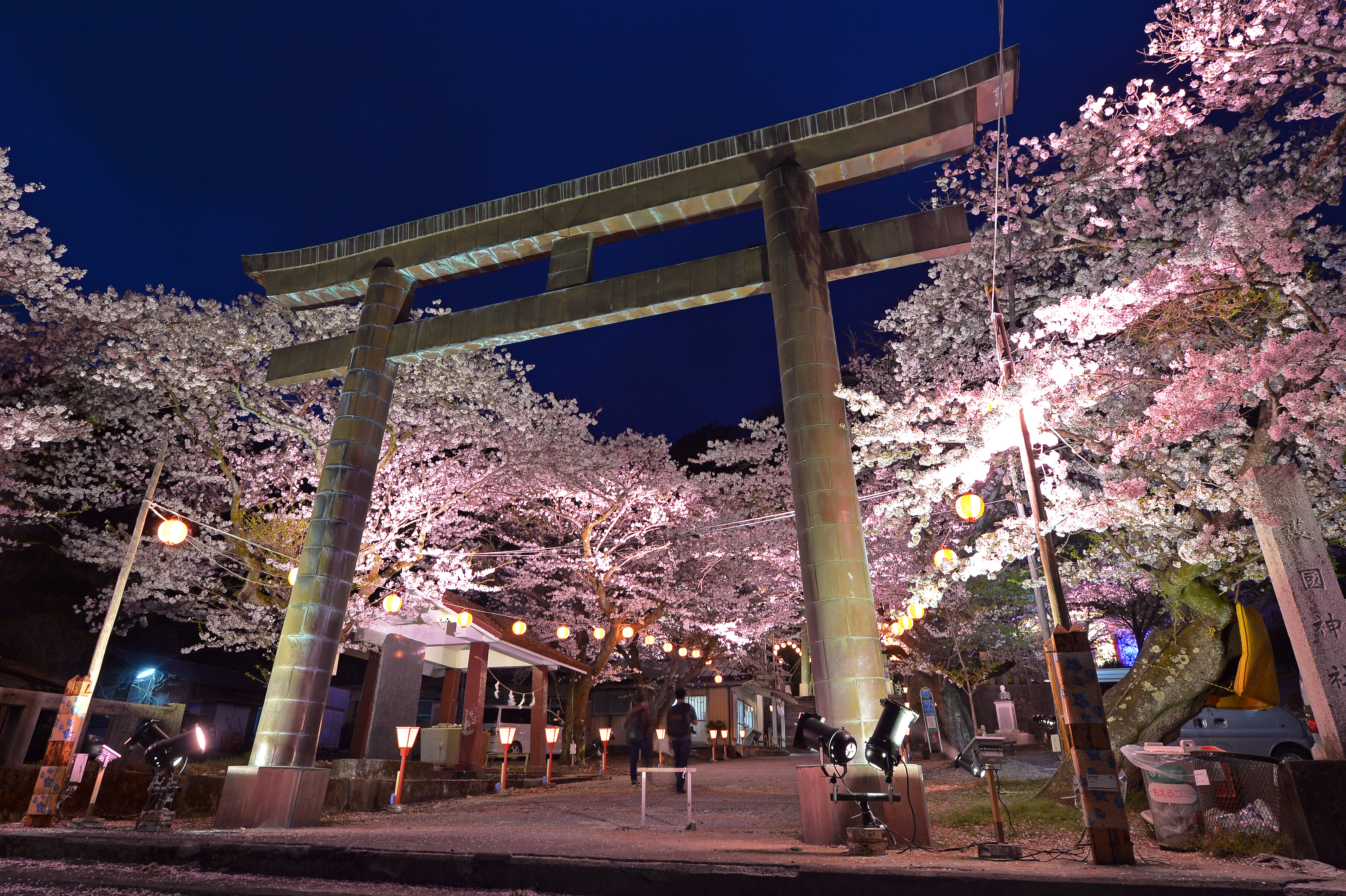The image captures a low-angle shot of a Japanese monument entrance at night, characterized by two large stone pillars that form a gateway. The pillars are a brownish beige color, and above them sits a horizontal column. This gateway introduces a path adorned with cherry blossom trees, identifiable by their pale pink blossoms, which are abundant and create a magical canopy. The scene is well illuminated by garden lights strung along poles, casting a warm orange glow. The rich, almost navy blue night sky enhances the tranquil and enchanting atmosphere, devoid of stars. A few people can be seen walking, adding a sense of peaceful human presence. The setting suggests a serene and picturesque location in Japan, possibly a Shinto temple, highlighting the traditional and inviting aesthetic of the scene.